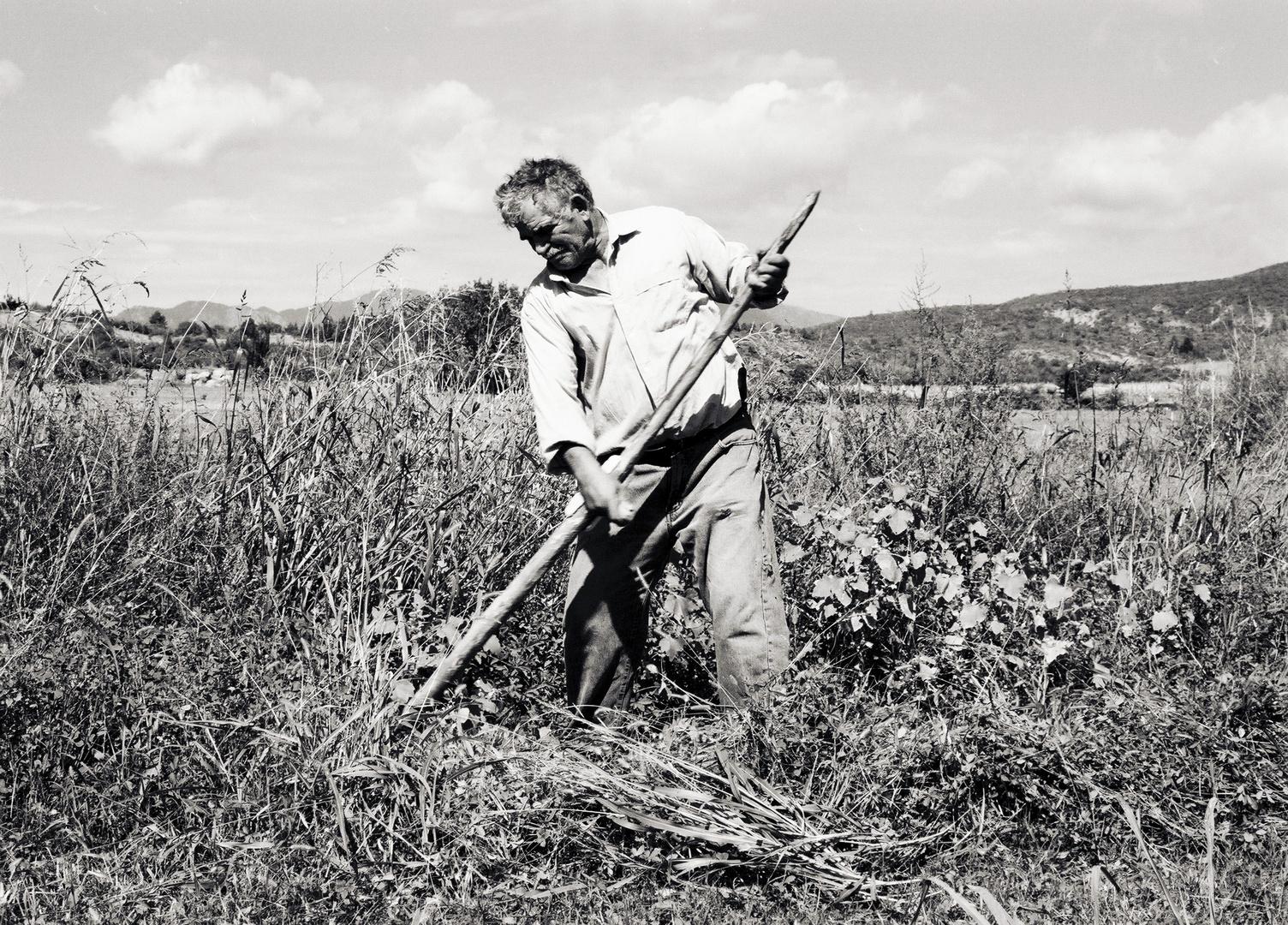This black and white photograph captures an elderly farmer laboring alone in his field. He is dressed in well-worn jeans, a loose fitting shirt with the sleeves rolled halfway up, and the collar unbuttoned. In both hands, he grips a wooden farming tool, though the specific implement is obscured by the dense vegetation surrounding him. The vegetation varies greatly in height, with some plants reaching up to his shoulders and appearing quite dried out. The farmer appears to be using sheer muscle power to clear the land, without any modern machinery to aid him.

The atmosphere is partly cloudy, casting a subdued light over the scene, which suggests a possibly arid climate. In the background, tall grasses, weeds, and flowers stretch across the field, indicating a long and overgrown season. The backdrop also features rolling hills and maybe even distant mountains, with cleared fields tucked behind the overgrown weeds, hinting at a larger homestead.

This image, which has an aged quality that suggests it dates back to the 1920s or 1930s, evokes a sense of hard work and resilience in challenging conditions.